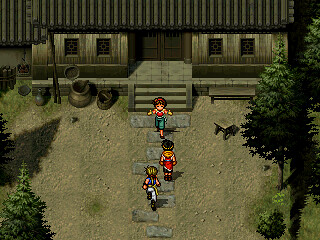The scene resembles a vivid and immersive setting from a video game, viewed from an elevated perspective. Beneath the tree canopy, a dirt and gravel lot is visible with a modest house positioned centrally. Stone steps are meticulously embedded into the ground, forming a walkway that guides the viewer to a gray wooden-frame house. The home's front porch is partially sheltered by a striped brown and white canopy, adding a touch of color and character.

In front of the house, the ground is sparse with various metal urns and miscellaneous items scattered around, contributing to the rustic ambiance. Two individuals are seen making their way up the stone steps towards the house, while a young girl stands at the foot of the stairs with her arms spread wide, welcoming them.

Flanking the gravel pathway, lush green trees add vibrancy and contrast to the subdued tones of the dirt and gravel. The entire scene is complemented by the intricate details, such as the graystone steps and the varied items outdoors, creating a realistic and engaging environment typical of richly detailed video game settings.